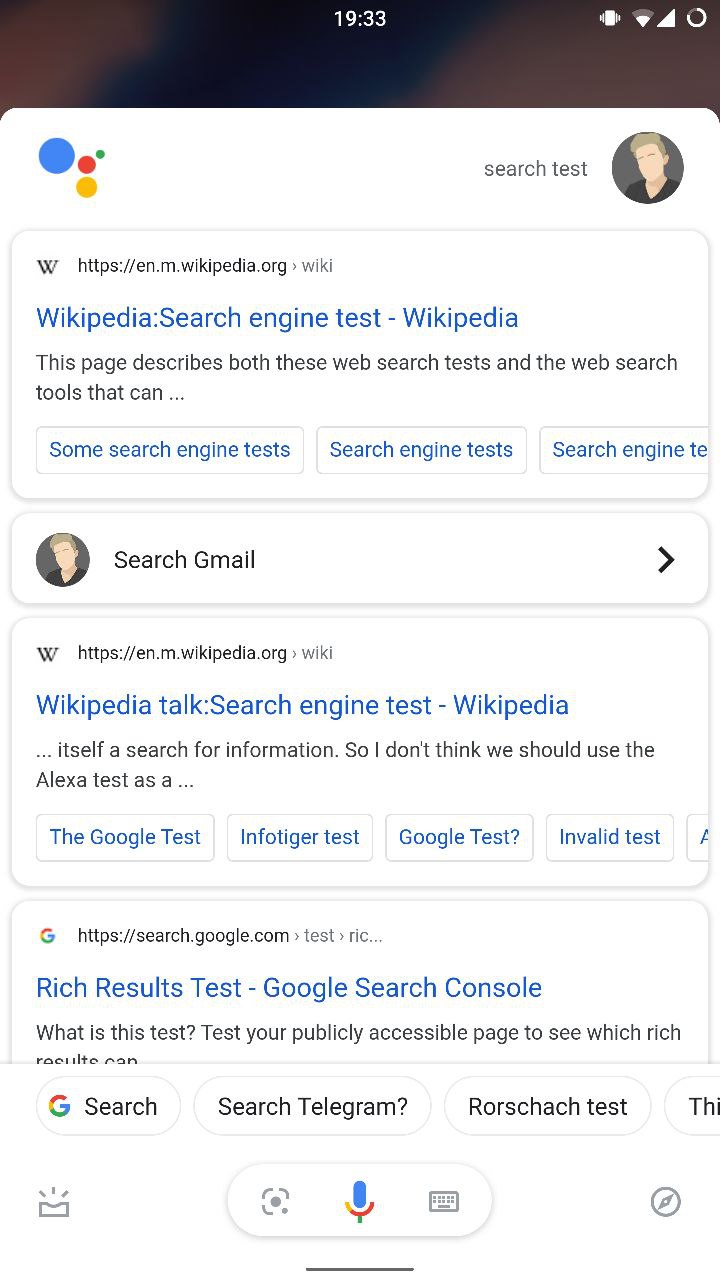**Detailed Screenshot Description:**

The image is a screenshot taken from a smartphone. The top inch of the screen features a gradient starting with a dark reddish color transitioning to black, and then back to dark reddish towards the center. In white text, the number "1933" is displayed prominently in the center-right area.

On the right side of the status bar, there is a circle with approximately three-quarters of it appearing white and the remaining quarter gray. The status icons show a full internet connection, Wi-Fi status at half strength, and a vibration icon.

Below the status bar, the background turns white. In the top-left corner, a large blue circle is visible, followed by a smaller red circle down and to the right of it, and a yellow circle beneath both. 

On the right side of this section, there is a profile picture of a cartoon character wearing a black shirt with brown hair and a black background. To the left of the profile picture, there appears to be a black search bar.

Underneath, a white rectangular section contains a wiki search bar at the top, with a black "wiki.org" logo. Below this, the text "Wikipedia search engine test - Wikipedia" is displayed in blue, followed by two lines of introductory information.

Aside from the text content, there are three blue-tabbed sections naming search engine options:
1. "Some search engines"
2. "Search engine test"
3. "Search engine te" (which is partially cut off).

Further down is another white rectangular section with the same cartoon profile picture in the top-right corner. To the right of this, the text reads "Search Gmail."

Below this, a larger rectangle again features the "wiki.org" branding and similar content. This time, the blue tabs are labeled with different test options: "Google test," "Info-to-juror test," "Google test and invalid test."

Lastly, at the bottom of the screen, another partial rectangular section is visible, displaying the tab "Rich results test - Google Search Console" in blue. Additional tabs below this include:
- "Search" (with a Google "G" icon beside it)
- "Search Telegram"
- "Rorschach test"
- "Rorschach test"

A final tab shows icons for voice input (mic), photo input (camera), and a small square symbol on the right end.